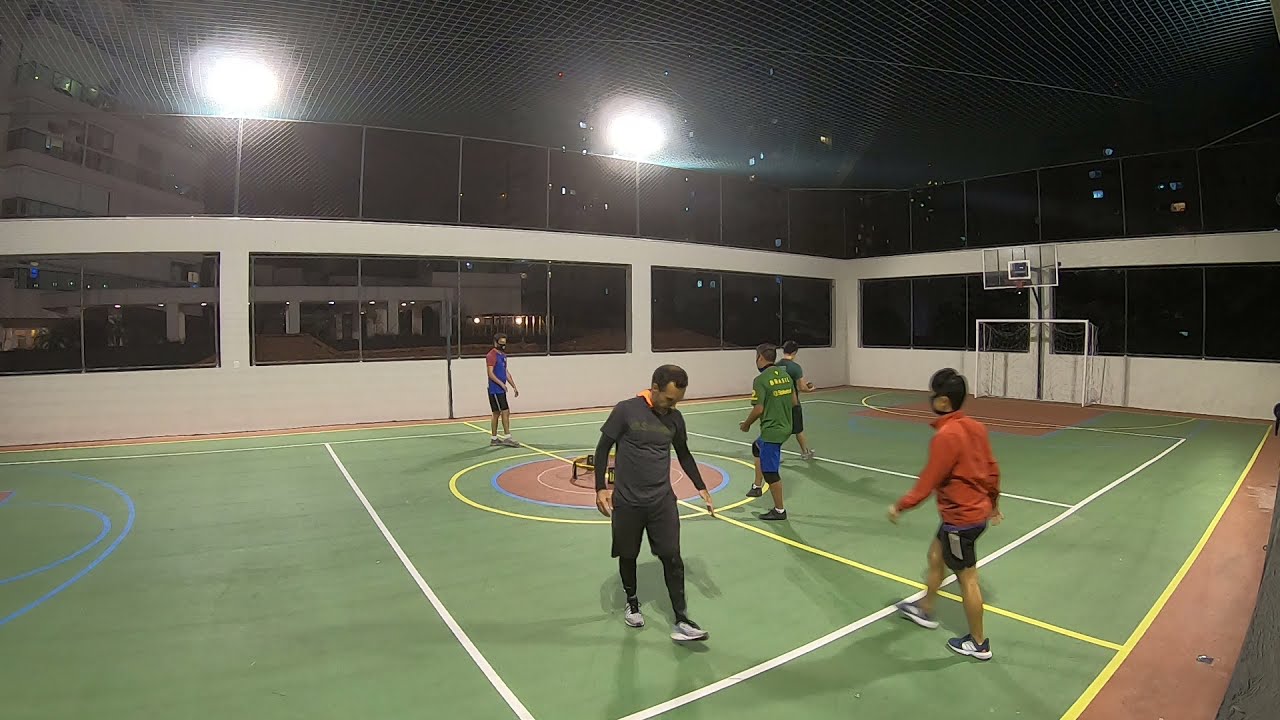The image captures an outdoor, yet covered, athletic court at night. The court is green with a colorful design that includes white and yellow lines and various circles, indicating it is multifunctional—likely used for basketball and soccer. The setting features white walls with large Plexiglass windows and a netted ceiling. There are five individuals on the court, engaged in athletic activity or possibly stretching exercises, moving in one direction. The participants are dressed in vibrant athletic wear—green, orange, black, and blue shirts, mostly paired with shorts and athletic shoes. Notably, there are visible basketball hoops on the right side of the court, adding to the recreational ambiance.